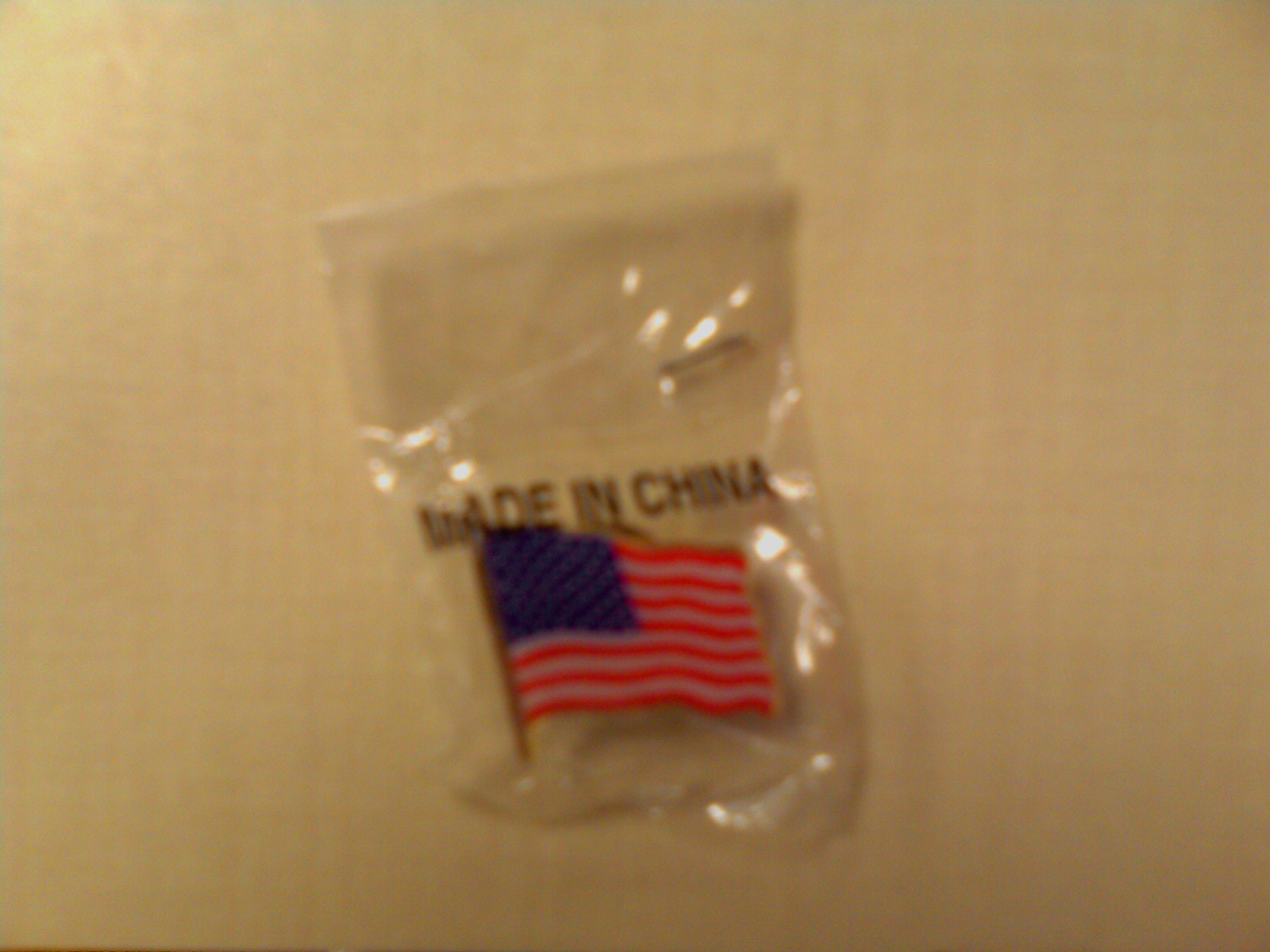The image is a color photograph featuring an extreme close-up view of an out-of-focus enamel pin depicting the Stars and Stripes of the American flag. The flagpole, positioned on the left side, extends downwards and appears to be gold, though the blurriness makes this detail ambiguous. The flag's dark blue canton occupies the top left corner and is rendered as a wavy rectangle, mimicking the movement of a flag in the wind. This blue section contains very tiny light spots, likely representing stars, though their precise shapes are indiscernible due to the focus.

The red stripes of the flag dominate the rest of the pin, with thinner gold stripes interspersed as substitutes for the traditional white. These red stripes appear bolder and striking against the gold-colored accents. The entire pin is encased in a clear plastic bag, with the text "Made in China" printed in black on the bag's surface. A small staple on the right side of the bag ensures the pin remains securely enclosed.